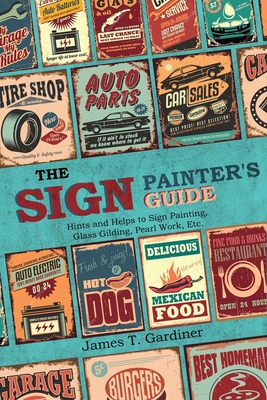This up-close photograph features a richly detailed decorative poster or book cover titled "The Sign Painter's Guide." The primary text, prominently featured in the center, reads, "The Sign Painter's Guide: Hints and Helps to Sign Painting, Glass Gilding, Pearl Work, etc." Above the main caption, there are several small, colorful portraits resembling miniature book covers or advertisements, including ones for "Auto Parts," "Car Sales," and "Tire Shop." Below the main title, more vibrant advertisements can be seen, such as "Delicious Mexican Food" with a chili and flame illustration, "Fresh and Juicy Hot Dog," and "Auto Electric." The author's name, James T. Gardner, appears just beneath these smaller images. The design includes a series of additional vivid depictions, each representing various businesses or services, like "Garage Burgers," "Best Homemade," and "Restaurant," all set against a sky blue background, creating a visually engaging collage.